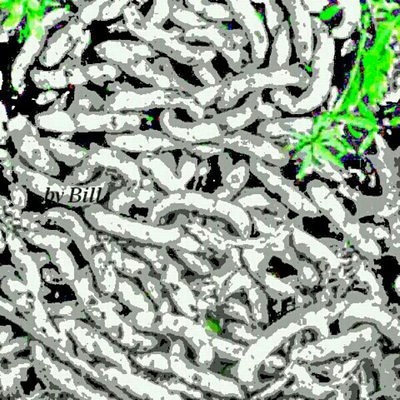This image appears to be a digital artwork by someone named Bill, featuring what looks like a chaotic mass of intertwined, worm-like shapes, primarily rendered in black, white, and gray. The twisting forms occupy the entire frame, creating a complex, swirling pattern that resembles either a clump of maggots or a microscopic view of bacteria. The image also includes sparse, vivid green touches: a small bit of greenery in the top left corner, another green element that appears leaf-like in the upper right, and a minor green detail at the bottom center. These green sections contrast sharply with the predominantly monochromatic palette. In the middle of the left side, there's a handwritten signature that reads, "By Bill," indicating the artist's identity. The overall piece has been edited to mimic a painted aesthetic, likely through photo manipulation software.